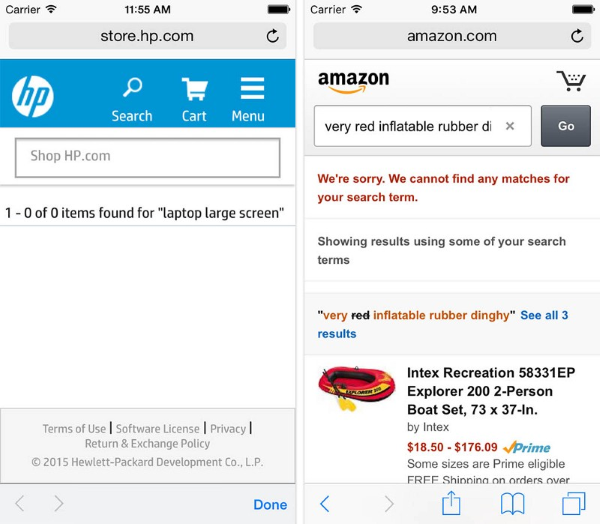**Dual Webpage Comparison: Detailed Analysis**

In this image, we observe two distinct webpage interfaces displayed on mobile devices, each showcasing different content and features. 

**Left Side: Hewlett-Packard (HP) Website**
- **Timestamp and Connectivity**: Captured at 11:55 AM with strong carrier signals and a full battery.
- **Website Details**: The HP website features a suite of navigation options starting with a search icon, a shopping cart, and a contact menu at the top.
- **Search and Shop**: Below these options, there is a search bar situated prominently, guiding users to search the site (shop.hp.com).
- **Content Display**: The page lists "large laptop" under the search results, along with various website footnotes including:
   - **Terms**: Terms of Use, Software License, Privacy, Return & Exchange Policy (2015).
- **Footer**: The page is concluded by a footer denoting Hewlett-Packard Development Co. LP with a "Done" button on the bottom-right corner.

**Right Side: Amazon.com Website**
- **Timestamp and Connectivity**: Captured earlier at 9:53 AM, also with a full battery.
- **Website Details**: The interface starts with the Amazon logo on the upper left and a shopping cart icon on the upper right.
- **Search Attempt**: The user searches for "Very Red Inflatable Rubber D." 
   - **Error Message**: The search term yields no exact matches, displaying an apologetic message and suggestions.
   - **Suggested Results**: Among the adjusted search terms, "Very Red Inflatable Rubber Dinghy" by Intex is highlighted:
       - **Product Description**: Intex Recreation 58331EP Explorer 200, a two-person boat set sizing 73 x 37 inches.
       - **Pricing**: Listed prices range from $18.50 to $179.09. Some sizes are eligible for Prime and offer free shipping on orders over a certain amount.
- **Footer**: The standard navigation and contact menus for Amazon.com are visible.

**Conclusion**: The side-by-side comparison demonstrates the differences in search functionality and user interface between the two sites. Notably, the Amazon search likely aimed for humor by posing as a request for a "Very Red Inflatable Rubber Dildo," a possible joke leading to the dinghy suggestion.